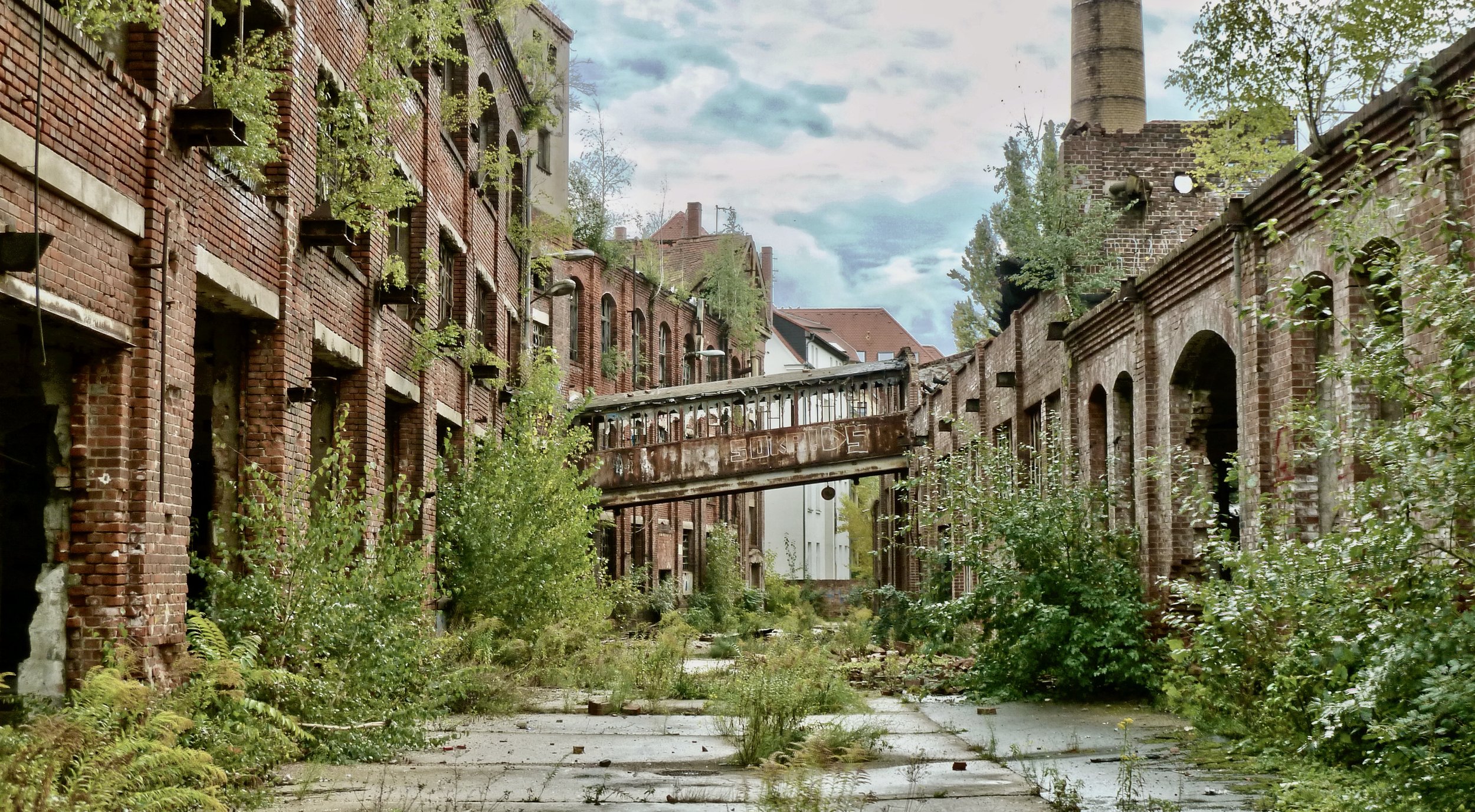The image depicts a thoroughly overgrown and abandoned urban scene. Dominated by a vivid blue sky with scattered white clouds, the photograph captures an old, neglected area featuring a concrete pavement overtaken by resilient weeds and tall grasses sprouting from the cracks. The central focus is a covered stone or concrete walkway that connects two buildings—one on the left made of brick and another on the right—forming a type of walkway bridge.

Flanking the walkway, a stone or concrete wall on the right has numerous arches, with more weeds and bushes growing densely around and on top of it. The buildings and the wall are framed by tall, weedy bushes, highlighting the overgrown nature reclaiming the space. The scene evokes a post-apocalyptic or abandoned city street atmosphere, blending elements that make it look potentially computer-generated, as might be seen in a video game background. The total absence of people further accentuates the desolate, neglected state of this setting.